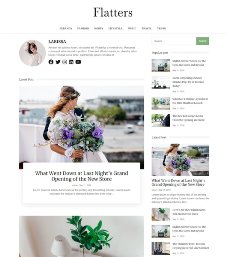This image appears to be a low-resolution screenshot from a blog or news website titled "Flatters." The top section features the website's logo and a menu bar with options that are indistinguishable due to the poor quality of the image. Directly beneath the menu bar, there is a small author profile image accompanied by a description, though it’s unreadable.

The main content begins with a prominent photograph that seems to capture a bride and groom, with the bride holding an elaborate bouquet composed of green and purple flowers. Below this image, there is a white rectangle that presumably contains the title and a brief description of the accompanying article, but the text is illegible.

The feed continues with another post, partially cut off in the screenshot, displaying only its upper section. On the right-hand side of the screenshot, there are thumbnail images for other posts, each paired with a title. However, the titles and images in this sidebar are also difficult to discern due to the image quality.